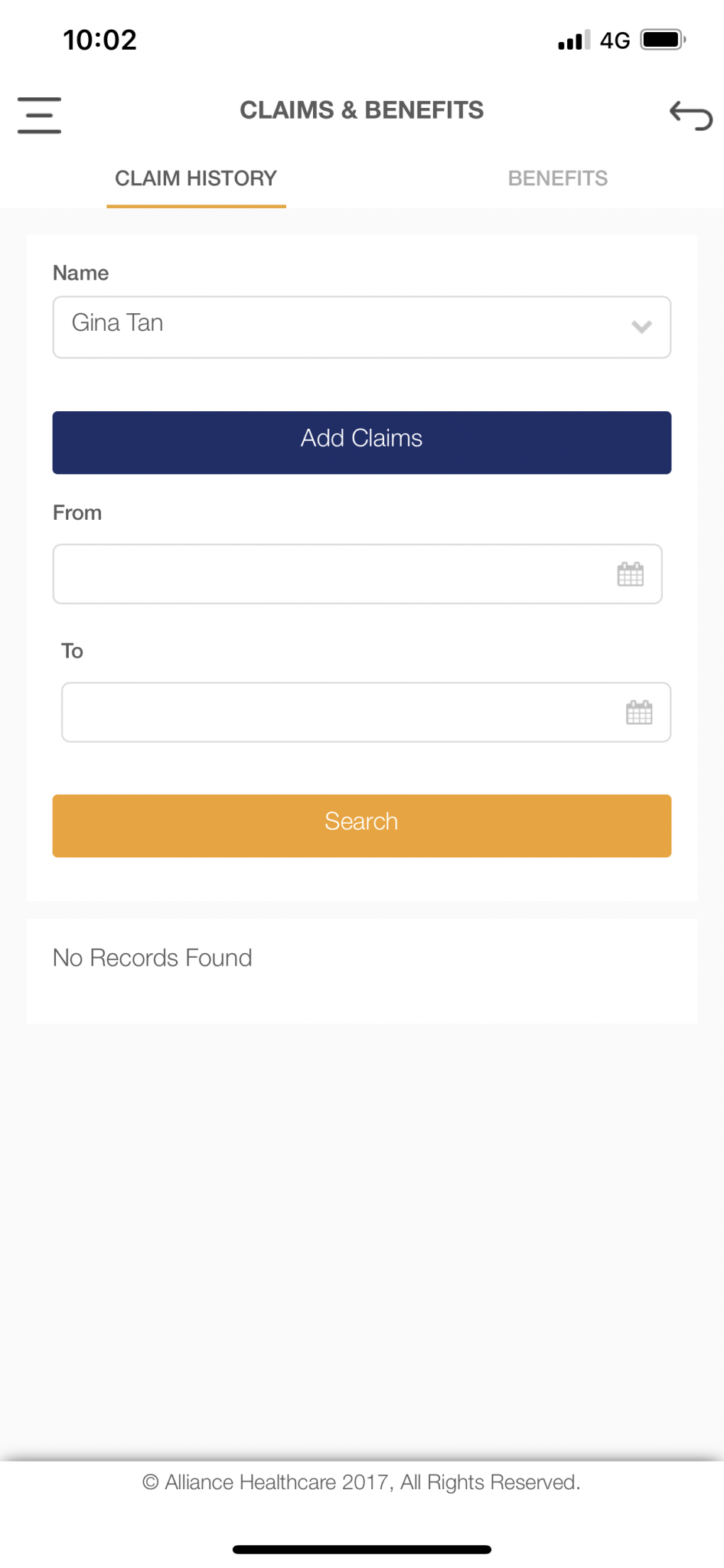The image shows a printout that appears to be a claims and benefit history page. In the top left corner, the number "1002" is displayed, and as you read across, a storage detail of "4 gigabytes" is noted alongside an almost full battery icon. At the top center, the title "Claims & Benefits" is prominently featured. Directly below this, "Claim History" is highlighted with a yellow underline, indicating its selected status, and the word "Benefits" is aligned to the right.

On the subsequent line, the name "Gina Tan" is entered. Following this, a dark blue bar with white lettering reads, "Add Claims." The next two lines contain fields labeled "From" and "To," both of which are empty. Beneath these fields, a gold bar with the word "Search" printed in white is displayed. The line below states "No records found," indicating that no data matches the search criteria. Finally, at the very bottom, a copyright notice reads, "© Alliance Healthcare 2017. All rights reserved."